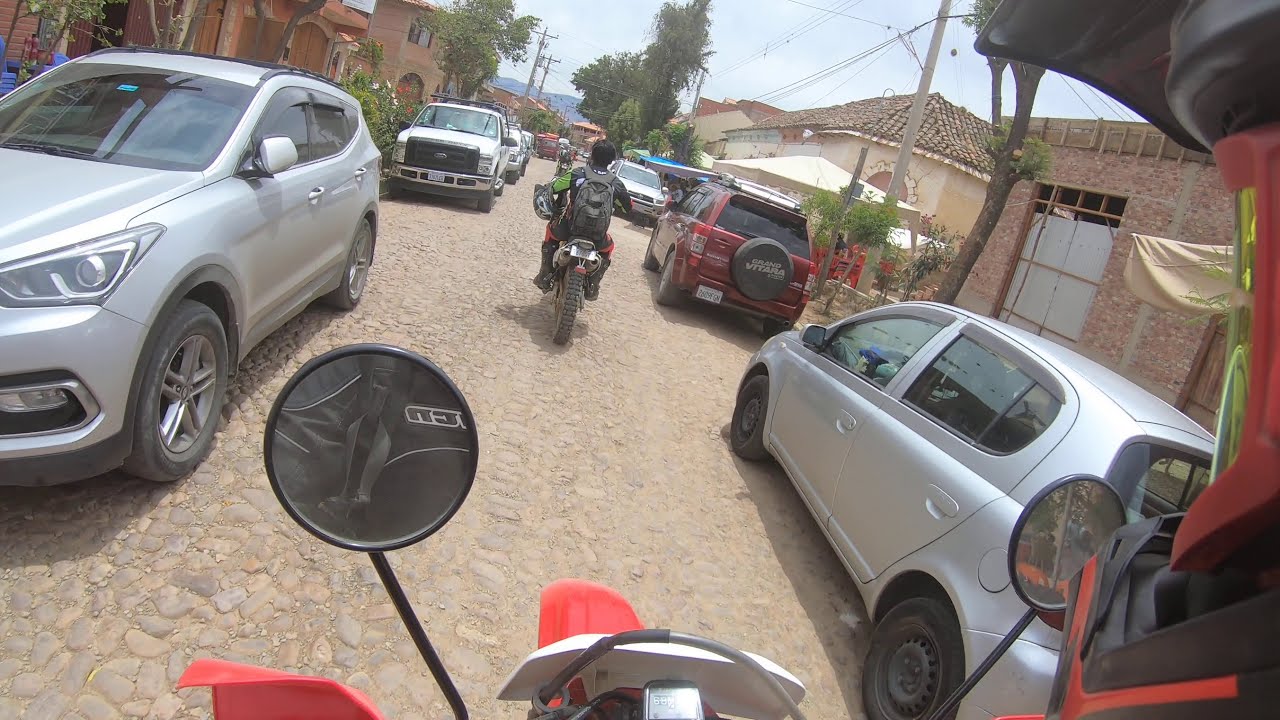The image depicts a narrow, light brown cobblestone street, likely in a small town or rural area, possibly in an Asian country. Cars are parked along both sides of the street, creating a congested thoroughfare. Among the parked vehicles, a silver boxy sedan can be seen on the right and another on the left, facing the viewer. A red SUV with a black tire mounted on the back is also parked along the street. In the middle of the road, a motorcyclist in full gear is riding away from the view. Additionally, the front end of another motorcycle, including mirrors and the front tire area, is visible at the bottom edge of the frame, suggesting the photo might have been taken from this vehicle. The buildings flanking the street are short, possibly constructed from stone or stucco, one featuring a tiled triangular roof. Telephone poles and electrical wires line the street, and trees can be seen in the far distance. The sky is bright and clear with a few faint clouds. The overall atmosphere is busy, with the street teeming with parked cars and motorcycles maneuvering through the narrow passage.